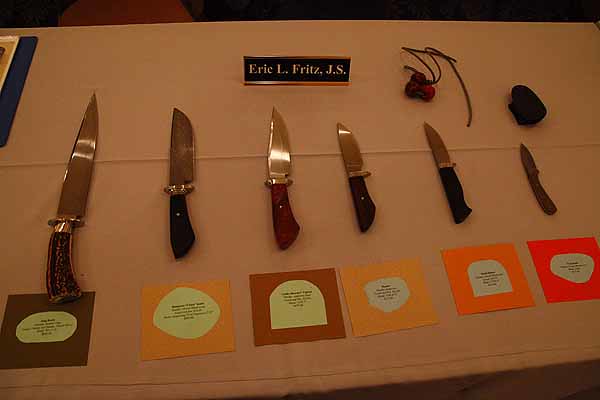This overhead image captures a dimly-lit presentation of six distinct knives meticulously laid out on a white table covered with a creased tablecloth. Positioned from left to right, the knives vary from largest to smallest, each identified by a colored card placed underneath the handle, featuring small black writing on white circles. The knives display a variety of handles—including bone, wood, and plastic—and diverse blade shapes, ranging from long and sharp to short and pointy. At the top of the image, a black rectangular nameplate with gold borders reads "Eric L. Fritz, J. S." In the background near the nameplate, there's an additional object with strings attached, possibly a sharpening stone. The tablecloth's poor lighting casts an orange-red hue over the scene, adding to the distinct presentation.